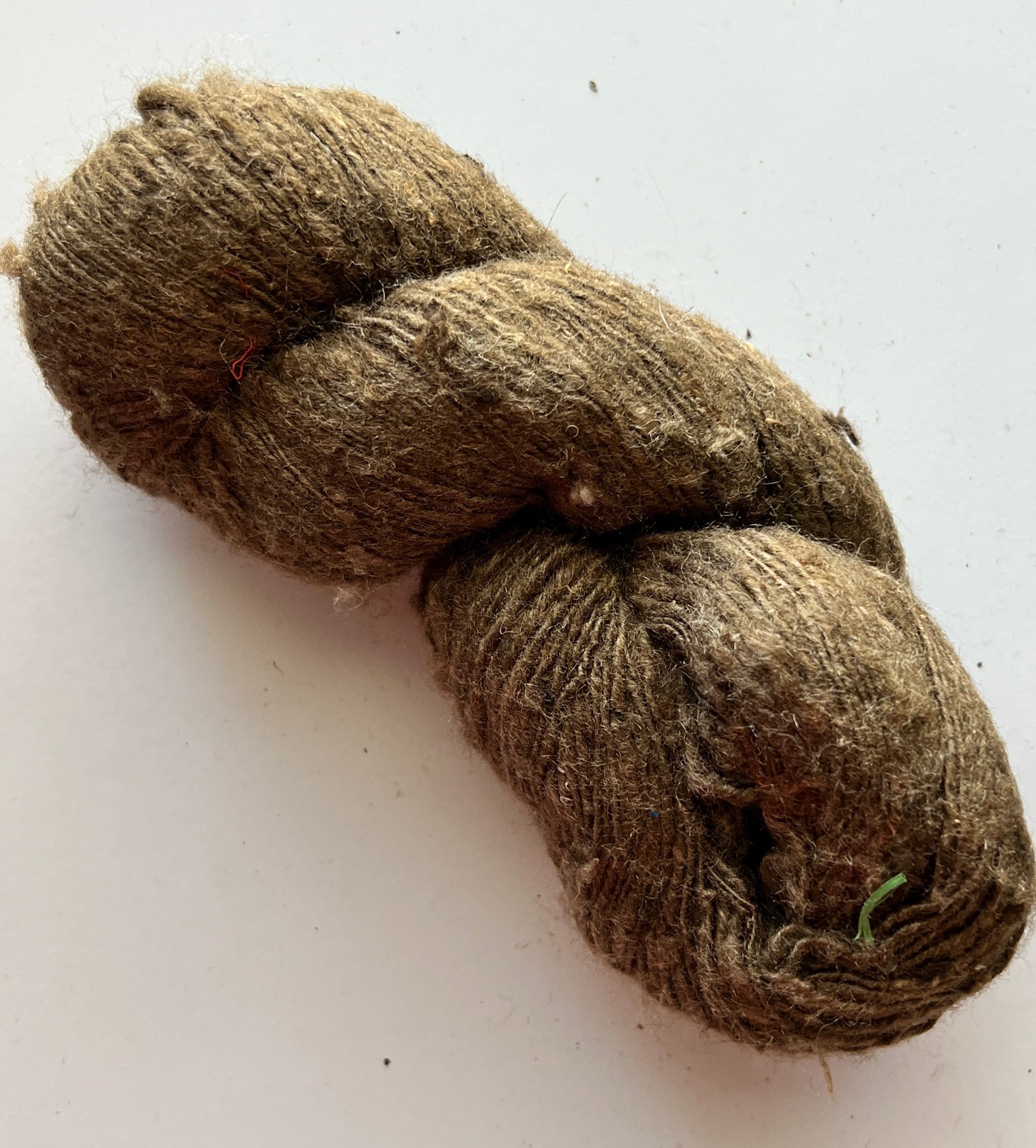The image depicts a mound of brown yarn that resembles a twisted rope or cocoon. The yarn is intertwined and fuzzy, with shades ranging from light to dark brown. Strands and threads are visibly extending from the main mass, which also shows signs of distortion and debriation. A notable detail is a small piece of green grass or string emerging from the bottom right-hand corner. The scene is set against a plain white countertop, and the yarn pieces have scattered slightly, dirtying the surface.